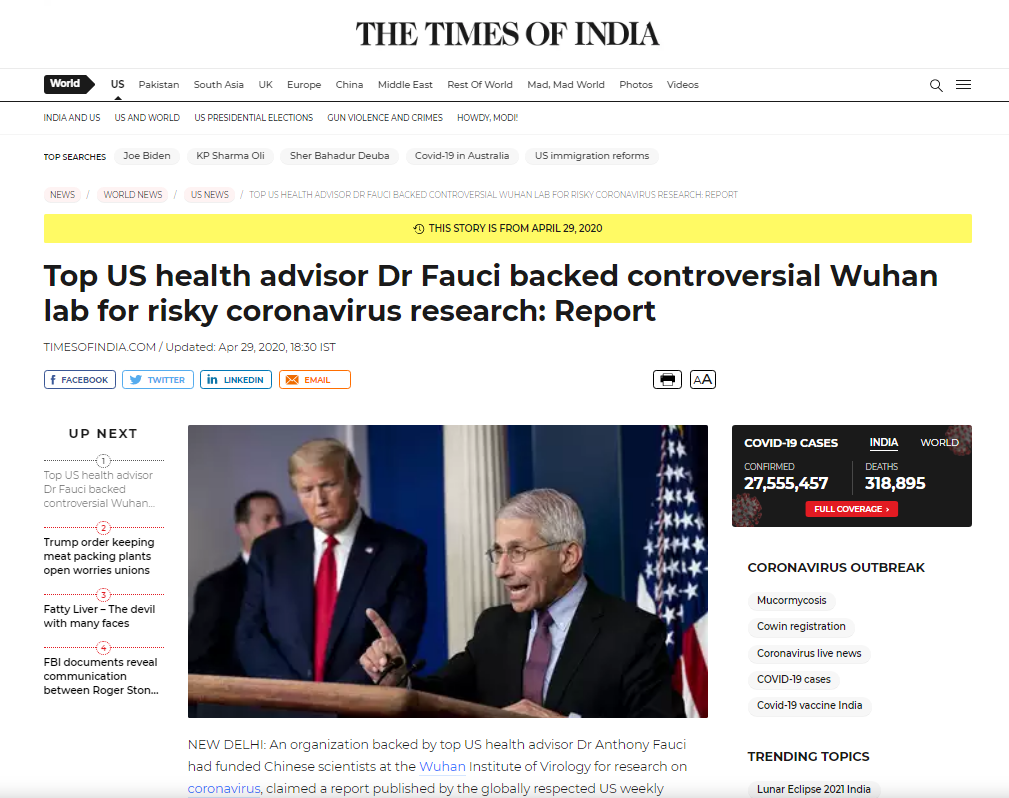A zoomed-in screenshot of the Times of India news website, magnified to 200%, features prominently on the display. The image captures the navigational section of the site, displaying various international categories in bold black text, such as "World," "U.S.," "Pakistan," and "South Asia," among others. The "U.S." section is selected, revealing a headline and a news image beneath. The headline reads, "Top U.S. Health Advisor, Dr. Fauci Backed Controversial Wuhan Lab for Risky Coronavirus Research: Report." The accompanying photograph shows Dr. Anthony Fauci at a podium, gesturing with his right arm extended, emphasizing a point as he speaks. To his left, former President Donald Trump stands attentively. Below the headline, a subheading states, "New Delhi: An organization backed by top U.S. health advisor, Fauci, had funded Chinese scientists at the Wuhan Institute of Virology for research on coronavirus," followed by additional text continuing the news story.